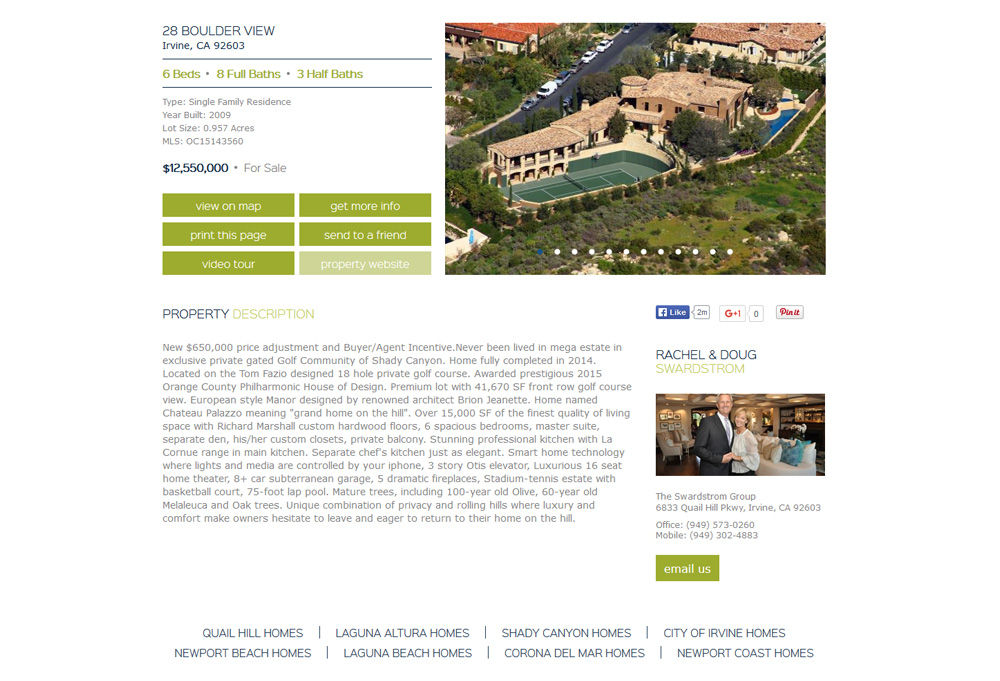**Overhead View of 28 Boulder View, Irvine, California 92603**

Welcome to the web page for the stunning property at 28 Boulder View, Irvine, CA 92603. This listing features an overhead photograph showcasing the expansive, beautifully landscaped property. The estate includes a large, elegant home surrounded by lush greenery, sprawling over a lot size of 0.957 acres. Built in 2009, this single-family residence offers 28 Boulder View's residents luxurious living with six spacious bedrooms, eight full bathrooms, and three half bathrooms. Additional amenities include well-maintained tennis courts.

The property is listed at a price of $12,000,000, with a detailed listing under MLS number OC15143560. For further details, the webpage provides six interactive tabs labeled: View on Map, Print this Page, Video Tour, Get More Information, Send to a Friend, and Property Website. Currently, the Property Website tab is active, which contains an extensive property description that is unfortunately too small to read from the image provided.

Under the property description, there are convenient share buttons for Facebook, Google+, and Pinterest. The page also features realtor information with a picture of Rachel and Doug Swardstrom from The Swardstrom Group. The image depicts them smiling warmly and standing chest-to-chest. Their office is located at 6833 Quail Hill Park, Irvine, CA 92603, with their phone numbers and email addresses provided for contact.

At the bottom of the page, there are additional navigation tabs for more property listings within various sought-after areas including Quail Hill Homes, Newport Beach Homes, Laguna Altura Homes, Laguna Beach Homes, Shady Canyon Homes, Corona Del Mar Homes, City of Irvine Homes, and Newport Coast Homes. This comprehensive listing offers a detailed glimpse into an exceptional property, expertly managed by the experienced Swardstrom Group.